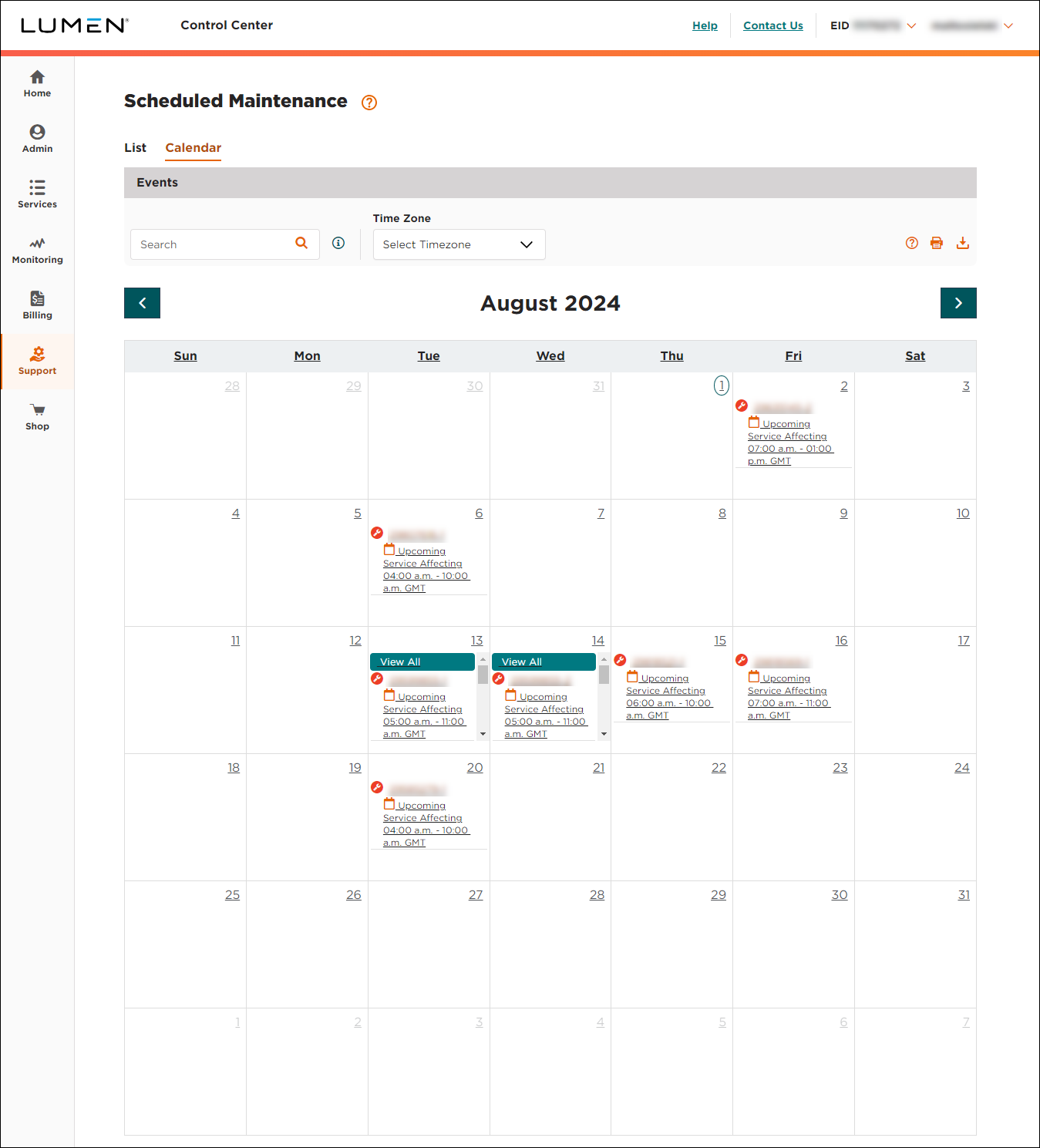The image displays an online calendar app interface. In the upper left-hand corner, the word "Lumen" is written in black, with the top of the letter "E" highlighted in blue. The background of the interface is white. On the upper right-hand side, there are partially obscured texts followed by visible options: "Control," "Centre," and "E, D." Below this, a blue horizontal bar spans the width of the interface with white text options on the right side, including "Explore Lumen," "Help," and "Contact us."

The left side of the screen features a very pale grey column housing several icons with accompanying labels. These labels include "Home," "Action," "Settings," and another, partly obscured, possible options such as "Messaging" or "Billing." Directly highlighted in blue is "Support," followed by "Shop."

At the top of the main section, there is a category labeled "Scheduled Maintenance" followed by "Manage Renotifications." Below this, the calendar navigation options include "List," "Calendar," with "Calendar" currently selected, and "Events." The interface also offers a search function specific to the calendar.

The detailed calendar displayed covers January 2023, with several dates featuring small, text-filled notifications. Due to the tiny text, these were difficult to read initially, so a closer look reveals the following details:

- On Tuesday, January 3rd, a notification reads "Completed service affecting 8am to 2pm GMT," accompanied by an icon of a tree encased in a little circle.
- On Wednesday, January 4th, another notification states "View all upcoming service affecting 6am to 12pm GMT."
- On Friday, January 6th, there's "Upcoming service affecting 5am to 11am GMT."
- Similar notifications are noted on the 10th, 11th, and 19th of January, each featuring a small round icon with a wrench symbol, indicating maintenance activities.

The meticulous details captured here provide a comprehensive view of the online calendar app's interface and scheduled events.